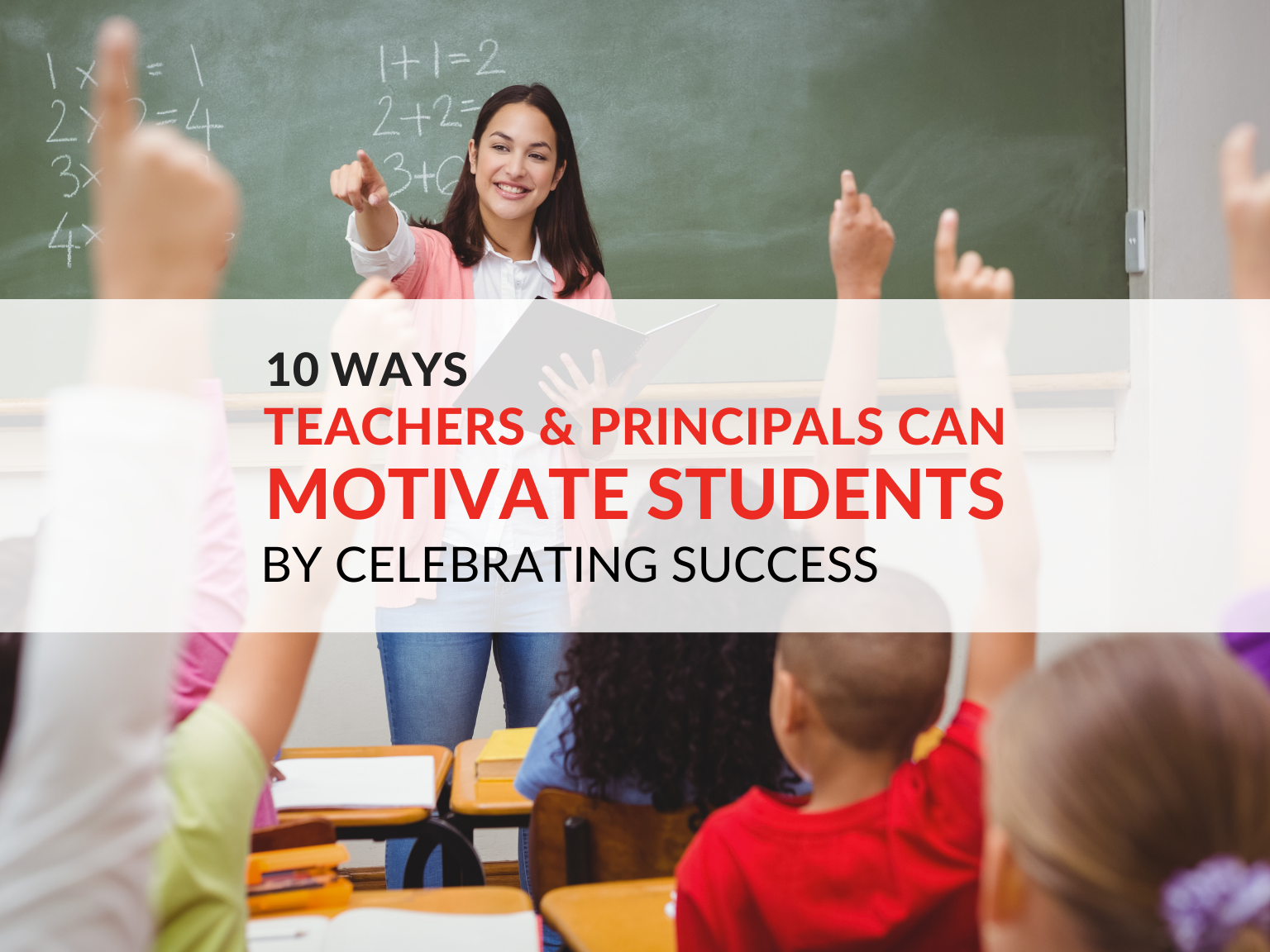The header image for the article features a vibrant classroom scene, showcasing a lively interaction between a teacher and her students. The teacher, possibly Latina, is dressed in a pink cardigan, a white button-up shirt, and blue jeans, with long brown hair cascading past her shoulders. She stands in front of a green blackboard adorned with simple arithmetic problems in white chalk, such as "1 + 1 = 2" and "2 + 2." Smiling warmly, she points towards a student while holding a book in her hand.

The foreground of the image captures the backs of several young students, ranging around five to six years old, seated at standard wooden desks. Enthusiastically engaged in the lesson, they have their hands raised eagerly, with visible diversity including a boy in a red t-shirt and several girls with long hair.

Prominently displayed across the middle of the image is a big white banner with black and red font that reads, "10 Ways Teachers and Principals Can Motivate Students by Celebrating Success," slightly translucent to allow the lively classroom atmosphere to peek through. This creates an inviting visual for readers to delve into the article's insightful content.